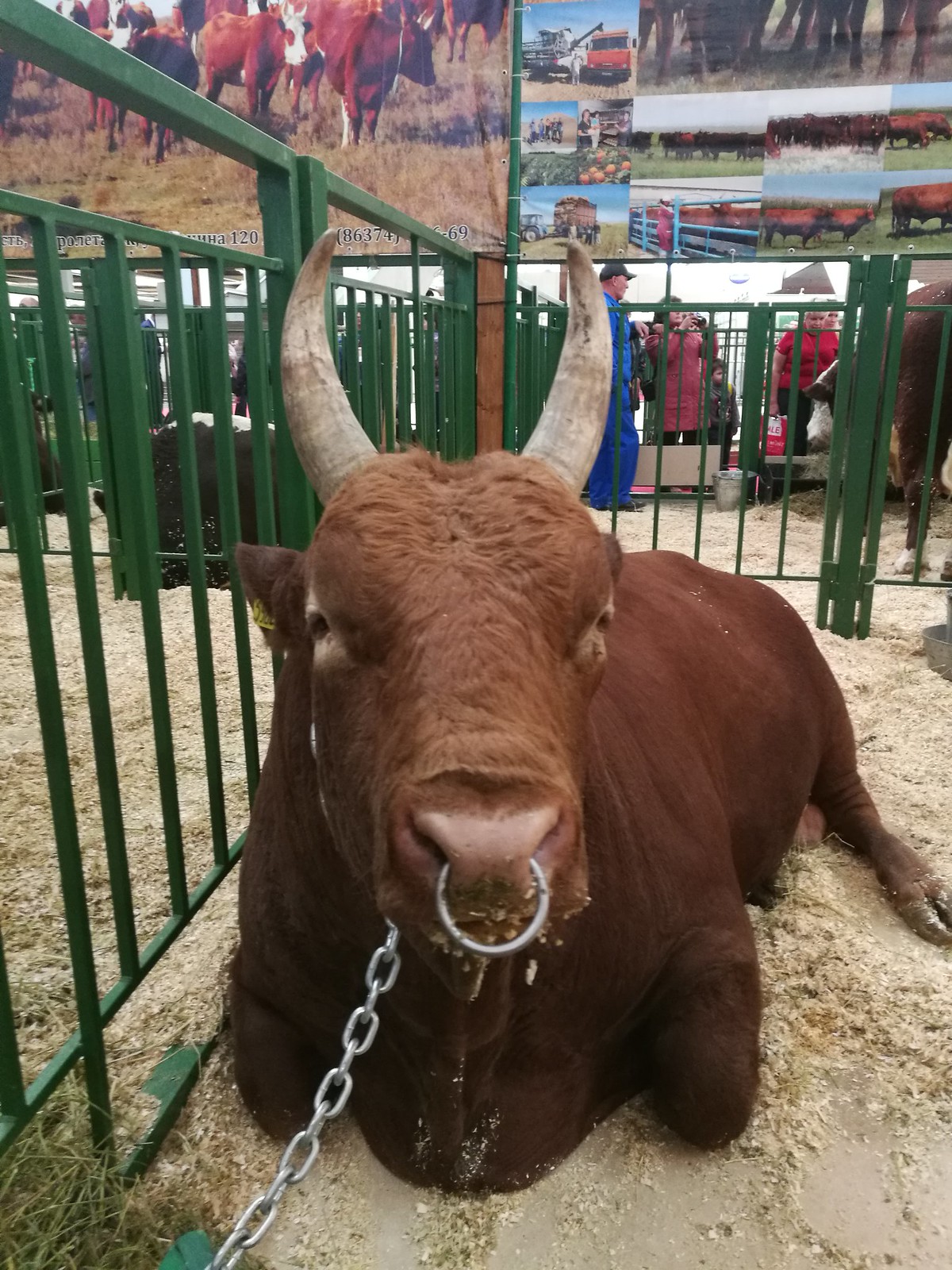The image features a young, chocolate milk brown bull reclining on a beige bedding, likely hay, inside an open-air barn. The bull, with a prominent silver nose ring and a thick silver chain attached to its neck, lounges peacefully within a fenced enclosure painted forest green. Its striking white horns, approximately two feet in length, curve slightly and add to its majestic appearance. Behind the bull, the background reveals another brown and white cow through the green metal bars and people milling about, including a woman in a red jacket and a man in blue wearing a hat. The setting is lively, suggesting a livestock event or bull riding show, with various enclosures housing more cattle. The enclosures are adorned with photos depicting ranch scenes and cattle, enhancing the rustic ambiance of the scene. A patch of green grass peeks from the bottom left corner, hinting at the animal's natural diet.